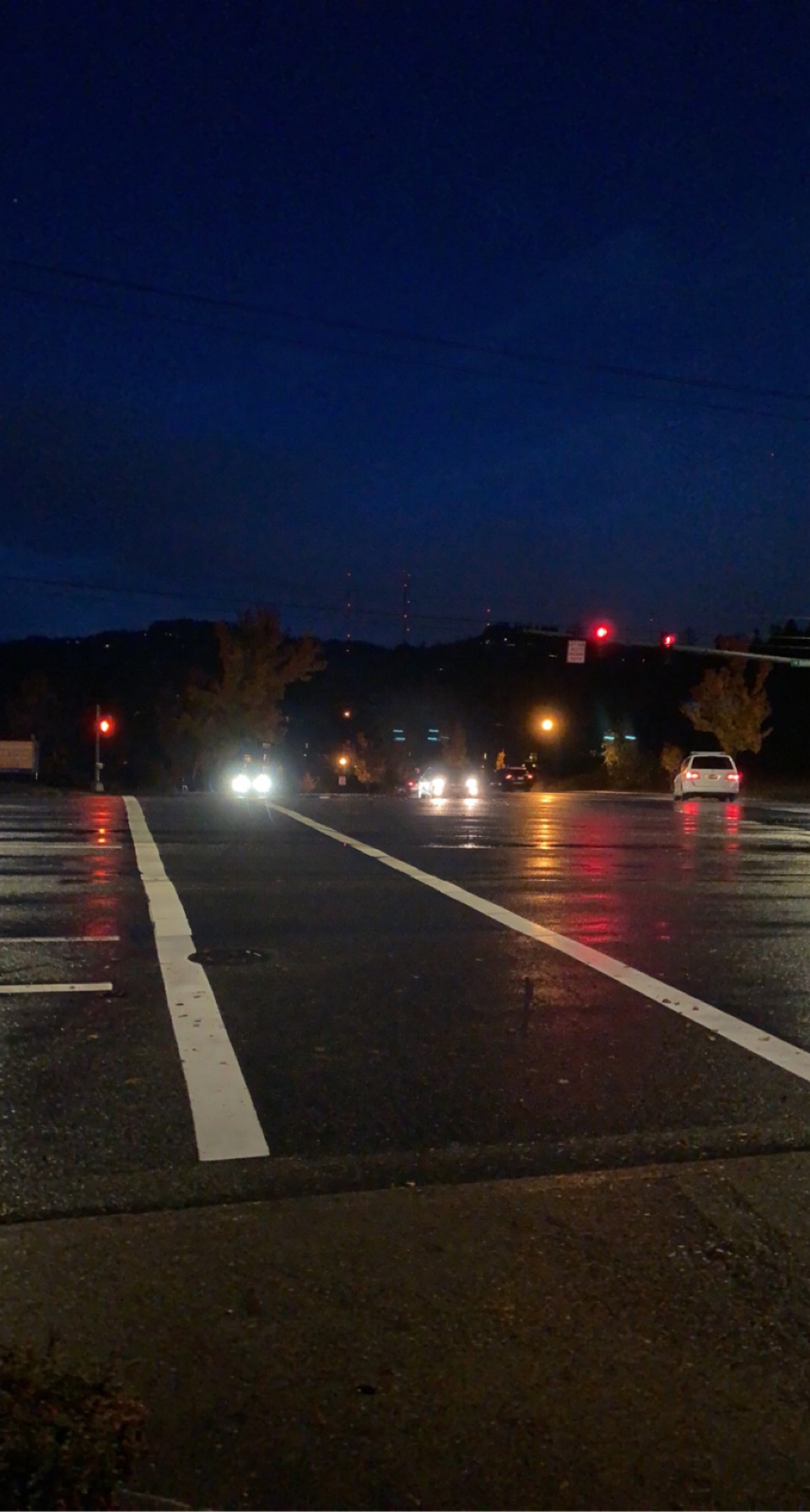Captured during the early evening, the sky is a serene medium blue, indicating twilight's arrival. The photograph is taken from the perspective of a sidewalk adjacent to a road. In the foreground, a pedestrian crossing is clearly visible with long white stripes stretching left and right. A manhole cover sits neatly within the walkway. To the left, a series of small white lines marks the parking spots, while to the right, the main roadway is in view. A few cars are seen up ahead, with two to three sets of headlights piercing the dusk. In contrast, the taillights of vehicles traveling in the opposite direction create a vivid red glow. A horizontal bar with stoplights spans the road, adding a sense of order and control. In the background, the imposing silhouette of mountains is visible, and several poles with red lights, used for airplane navigation, punctuate the skyline, adding a touch of modernity to the scene.